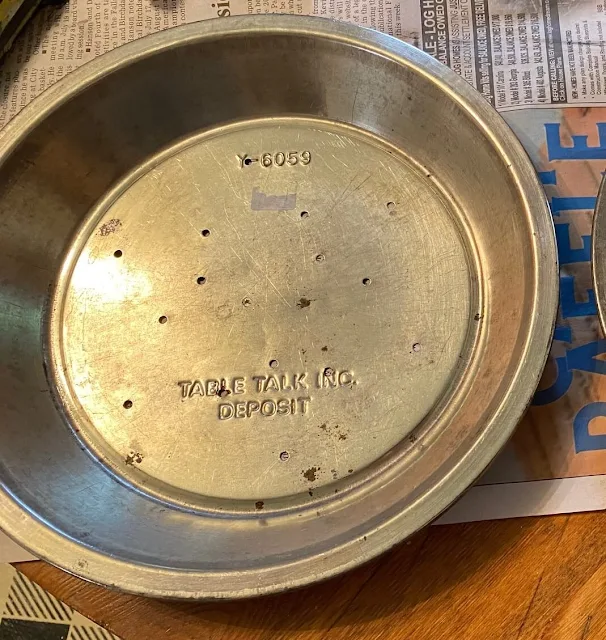The image captures a detailed overhead view of an old, silver metal pie pan, likely made from aluminum, resting on a newspaper that covers part of a light green-brown wooden table. The pie pan, which resembles a slightly weathered dog bowl, is the central focus and takes up most of the frame. It shows signs of age and use with noticeable corrosion, dirt, and scratches. Numerous small, seemingly random holes are stamped into the bottom of the pan. Stamped text on the inside surface of the pan reads "Table Talk Incorporated Deposit" at the bottom center, and "Y-6059" towards the top, resembling a serial number. Another pie pan's edge is faintly visible nearby, sharing the same wooden table surface.